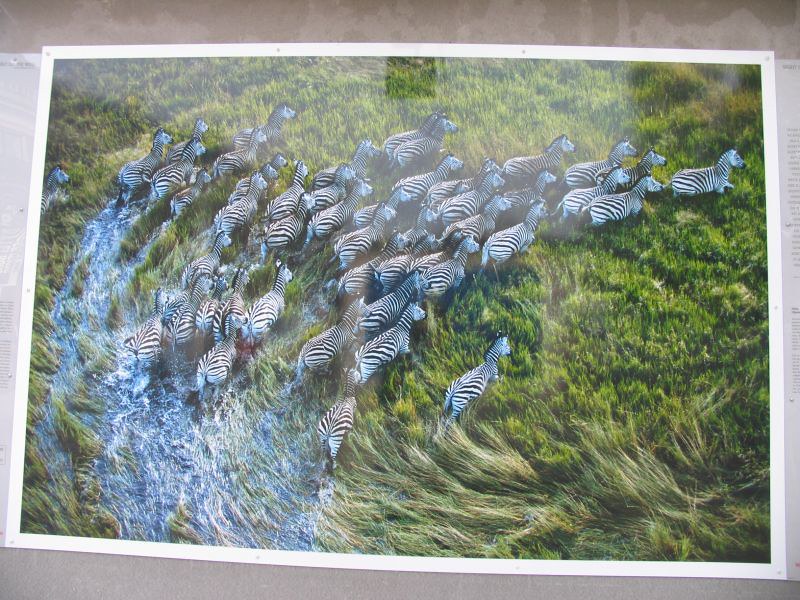The image is of a printed photograph inside a white frame, lying on a flat surface that appears to have a book or paper with printing to the right, and a table surface with a mix of tan, brown, and off-white hues. The photograph itself is an aerial shot capturing a herd of zebras numbering in the dozens, running in a dynamic arc from the left towards the right of the image. The zebras are mostly standard black and white, but the glare from the glass frame lends some of them a bluish tint, adding an unusual visual element. They are running through a grassy landscape with varying shades of green and amber, and part of the scene includes water merging with the grass, giving the impression of zebras rushing through a blend of land and water. Wind lines are visible, enhancing the sense of movement and flow across the field. The glare from the glass makes it challenging to focus sharply on all details, creating a reflective effect.